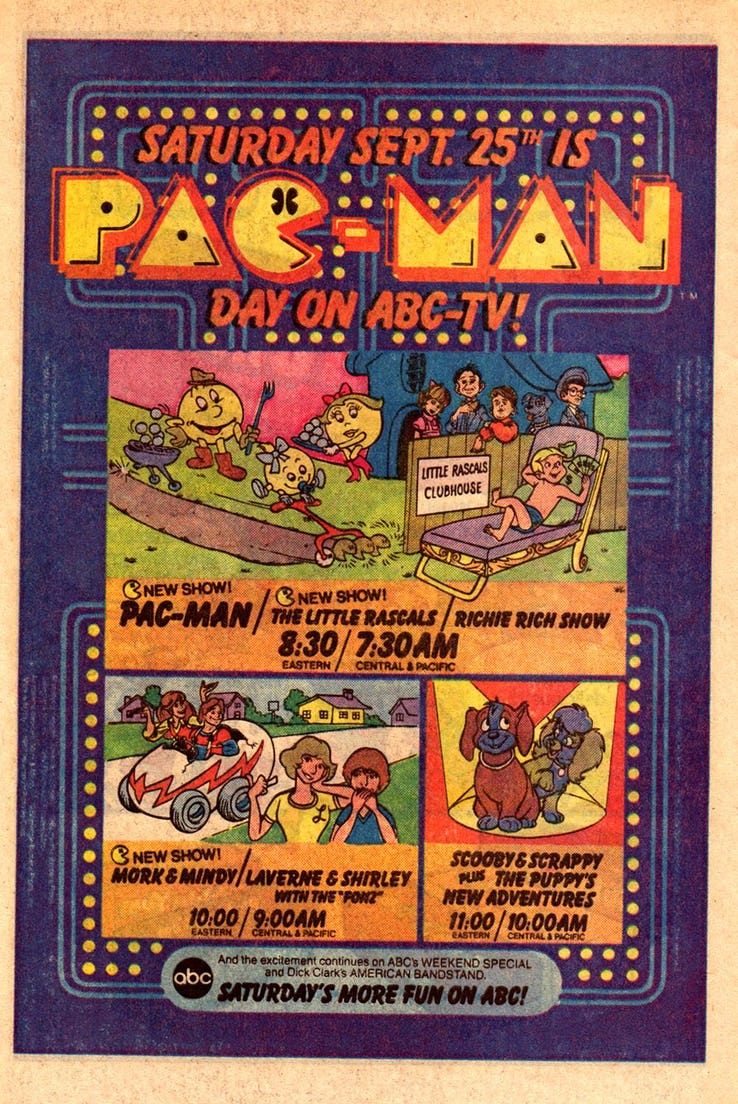This advertisement, likely from a magazine or TV guide, heralds "Pac-Man Day" on ABC TV, scheduled for Saturday, September 25th. At the top, in vibrant orange and yellow text, the announcement reads, "Saturday September 25th is Pac-Man day on ABC TV," set against a blue background reminiscent of a Pac-Man game maze. The central feature showcases the Pac-Man family, including Mrs. Pac-Man, Pac-Man, and their baby, engaged in yard work or grilling activities. To the right, children can be seen, with one child lounging in a chair and waving a fan of cash, set against a backdrop featuring a fence labeled "Little Rascals Clubhouse."

Above this scene, a banner highlights the new shows: "Pac-Man" and "Little Rascals." The ad also provides TV scheduling details: "Richie Rich" at 8:30 a.m. Eastern / 7:30 a.m. Central and Pacific. Below this, there's an advertisement for the new show "Mork & Mindy and Laverne & Shirley with The Fonz," slated for 10 a.m. Eastern / 9 a.m. Central. The lineup concludes with "Scooby and Scrappy-Doo and The Puppies’ New Adventures" at 11 a.m. The phrase "Saturday's more fun on ABC" punctuates the bottom of the ad in bold black text, summarizing the excitement of the animated Saturday lineup.